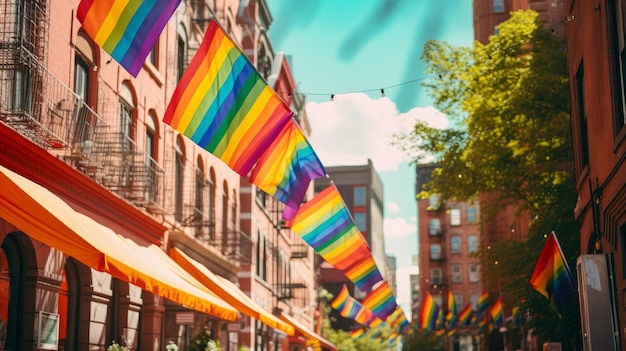The photograph captures a vibrant city street adorned for what appears to be a pride celebration. On the left side, there is a row of tall, brick buildings reminiscent of Brooklyn architecture, complete with windows and orange awnings above the entrances. Among them is a distinctive pink building, likely an apartment complex with a balcony. The right side features more brick structures and a prominent green tree that stands out in front of shadowed buildings. The sky is a striking blue, with a peculiar visual of a string or clothesline that stretches between buildings, possibly an artistic illusion.

Dominating the cityscape, numerous rainbow flags in a repeating pattern of red, orange, yellow, green, blue, darker blue, darker green, medium green, yellow, orange, red, pink, and purple hang overhead. These flags extend across the entire photo, lending a festive atmosphere and emphasizing the celebration of pride. The vivid and extensive display of these flags suggests a special event or festival in honor of LGBTQ+ pride.